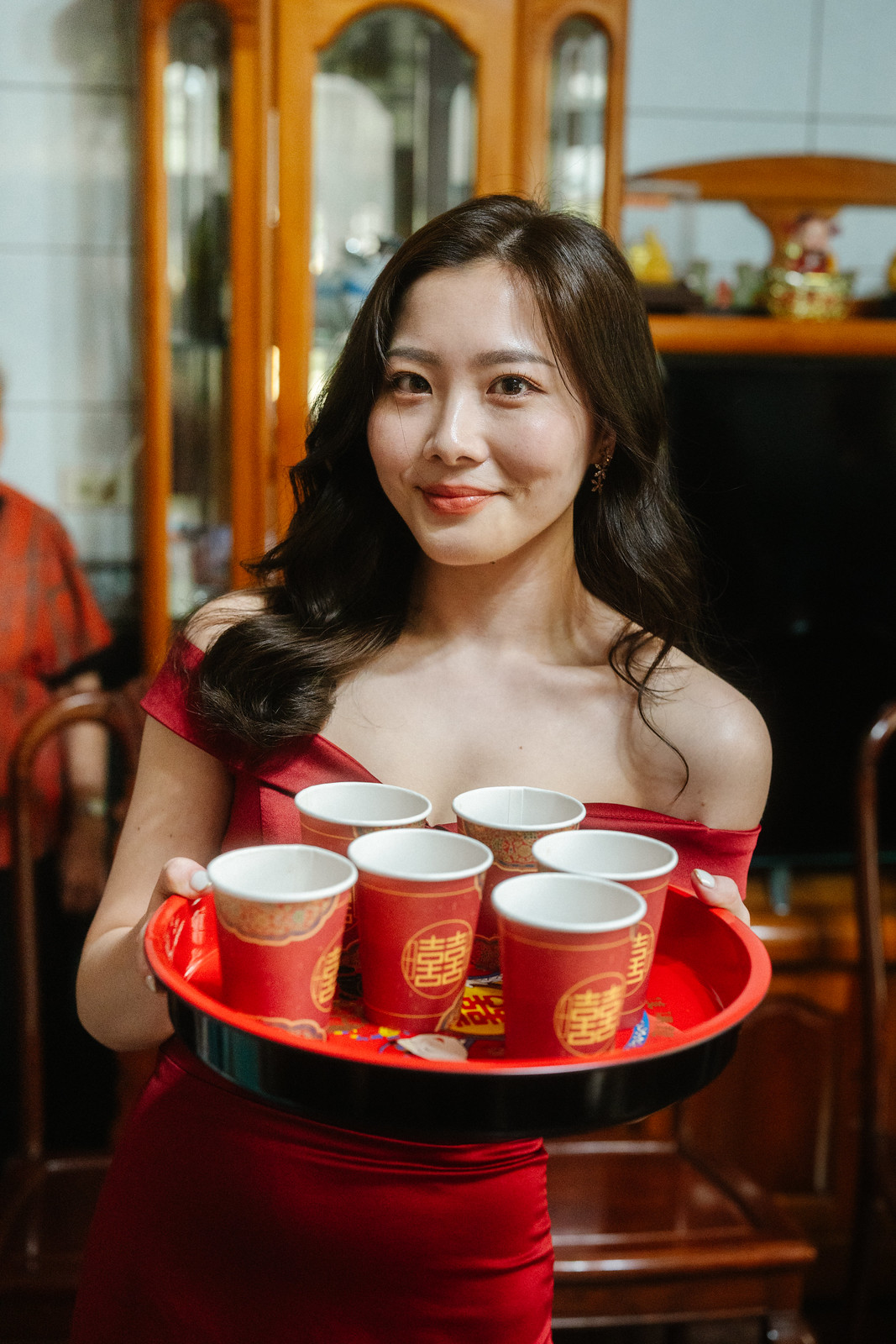This color photograph captures a beautiful young Asian woman, possibly Chinese, with shoulder-length, wavy, dark brown hair parted in the middle. She is adorned in a tight-fitting, off-the-shoulder red satin cocktail dress that elegantly showcases her neckline and shoulders. With a warm, closed-mouth smile, she extends her arms towards the camera, presenting a large, round, red serving tray. The tray is predominantly black on the outside and red inside, featuring a golden Chinese emblem in the center. Arranged neatly on the tray are six red paper cups, each embellished with a gold circular design and Chinese characters.

In the background, which is blurred to keep the focus on the woman, we can faintly see a mixture of black and orangish-brown wooden furniture, including a china cabinet with three tall, arched glass doors filled with knickknacks and trinkets. Additionally, there are wooden chairs and tables suggestive of a restaurant setting. Notably, to the far left, a partial figure of another person is visible, identifiable by their red shirt and wristwatch, adding a subtle dynamic element to the scene.